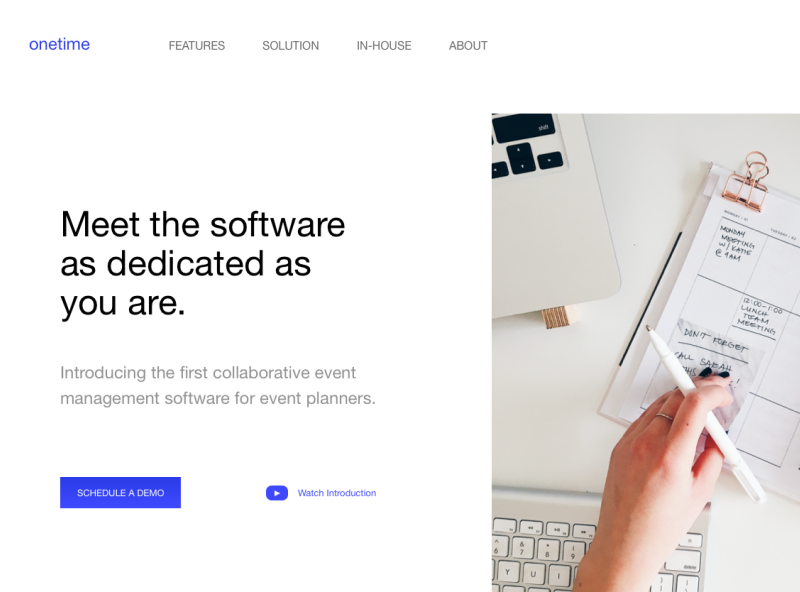A top-down view of a white desk featuring a screenshot of a website homepage for a software dedicated to event planners. On the left side of the screenshot, the hero text reads, "Meet the software that's as dedicated as you are," indicating the software's focus on collaborative event management. On the right side, a Macintosh wireless keyboard and a Mac Pro on a kickstand are visible. A woman, holding a white pen in her left hand, is interacting with a calendar that has a paperclip attached to it, while also handling a Post-it note. Below the hero text, there are options to "Schedule a Demo Call" and "Watch Introduction," both highlighted in purple with a YouTube play icon next to the introduction option. The logo for the software, "One Time," appears in the upper left, also in purple, flanked by navigation options: Features, Solutions, In-House, and About. The background is entirely white, emphasizing the clean and minimalist design of the homepage, aimed at encouraging visitors to explore the demo or sign up for the service.